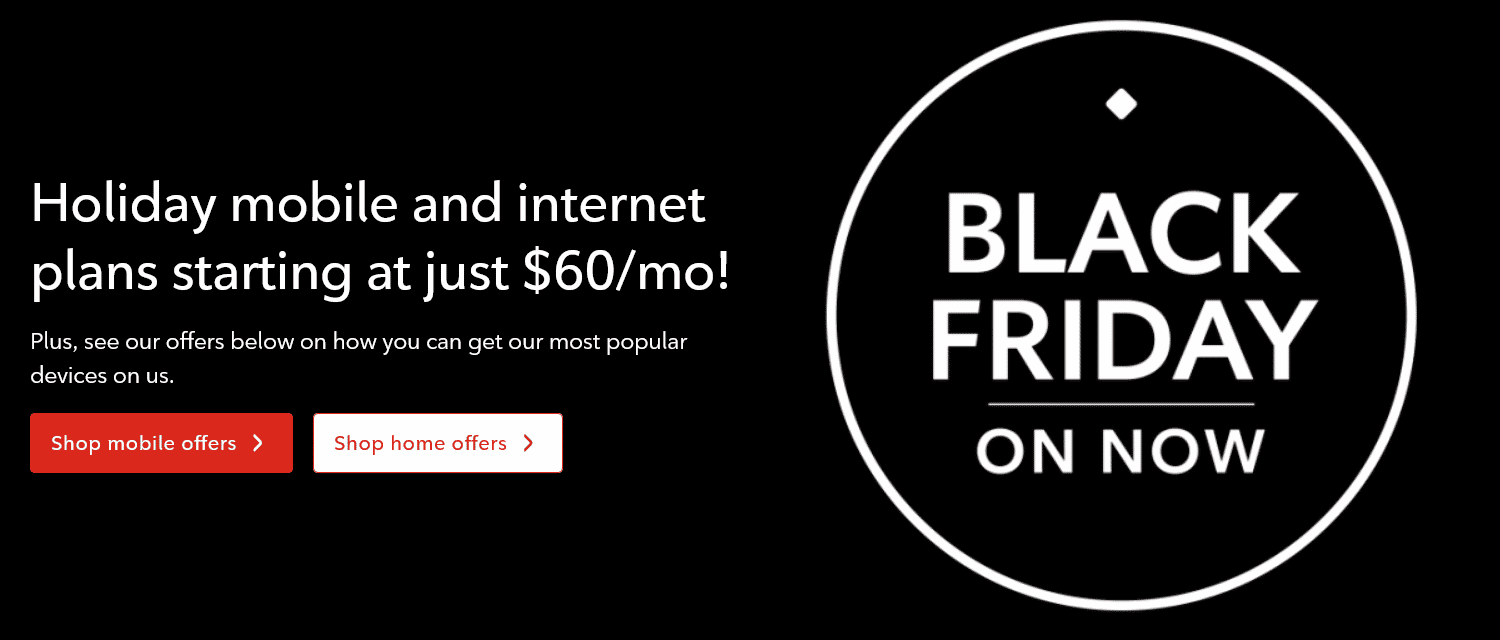The image features a stark all-black background. On the right-hand side, there is a prominent white outlined circle. Within the circle's center, a tiny white diamond is positioned towards the top, with "Black Friday" written directly beneath it in large, bold letters. Below the words "Black Friday," a white line is drawn, under which the phrase "On Now" is neatly presented.

Towards the left side of the image, white text is prominently displayed. The larger font reads: "Holiday Mobile and Internet Plans Starting at Just $60/MO!" In smaller text below, it states: "Please see our offers below on how you can get our most popular devices on us."

Additionally, there are two call-to-action buttons within the image. The first button, a red rectangle, is situated towards the bottom-left area and contains white text that reads "Shop Mobile Offers," accompanied by a greater than sign (>). To its right, another button is illustrated, this time in white with red text that says "Shop Home Offers," also featuring a greater than sign (>).

The overall layout is minimalistic, focusing on the high-contrast black background and white text accents, with bursts of red in the call-to-action buttons. The black background ensures the white text and red elements stand out strikingly for maximum visibility and impact.